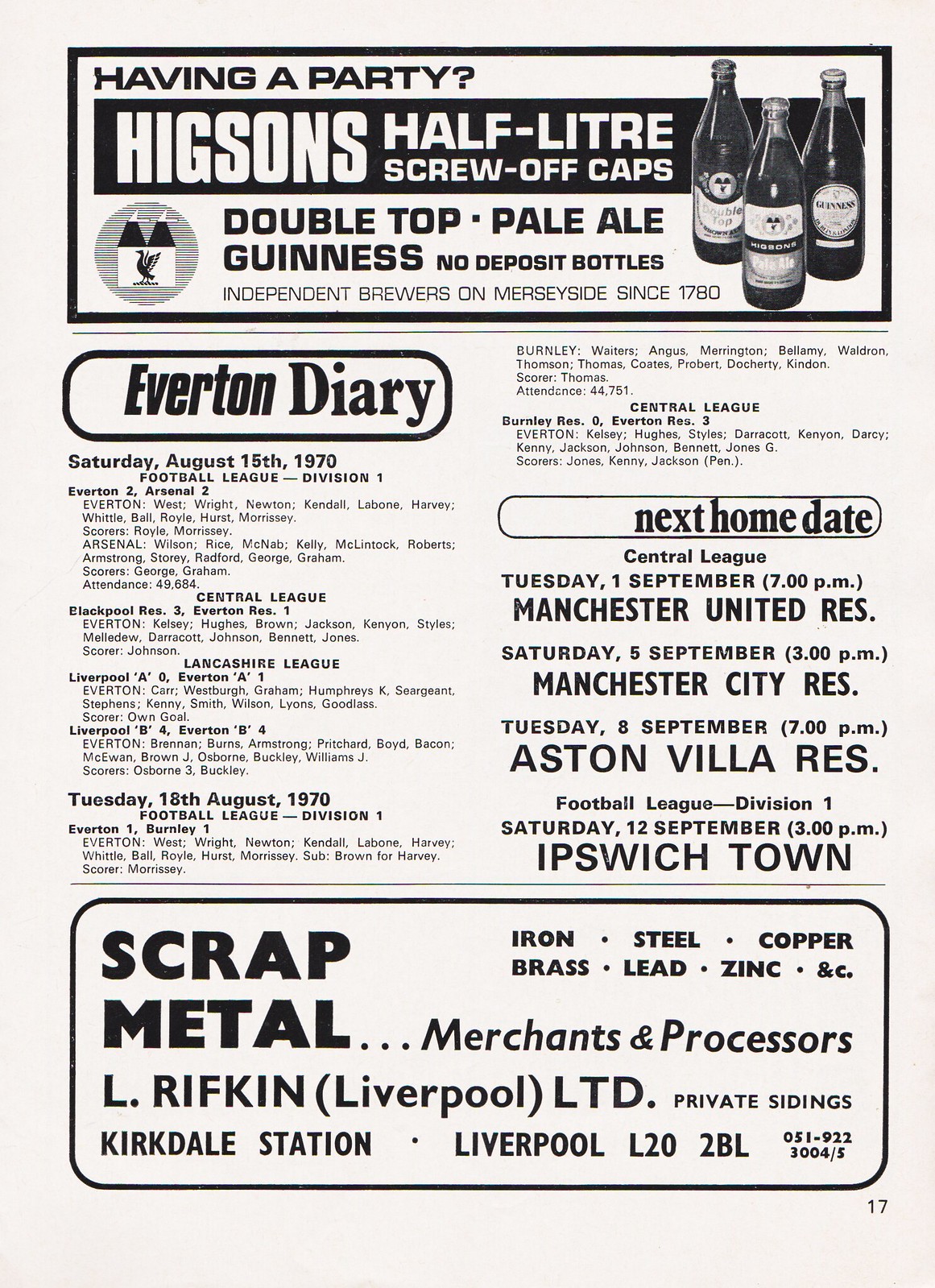The image shows a black and white page, likely from a local newspaper or soccer program dated 1970. The upper quarter of the page features an advertisement for Higgins Half-Liter Screw-Off Caps Double Top Pale Ale Guinness, produced by independent brewers on Merseyside since 1780. The ad displays three bottles on the right and a bird-like emblem in a circle on the left, with a header tagline "Having a party" above.

Below this ad, the main content of the page, divided into two columns, details various soccer matches. The left-hand column, labeled "Everton Diary," lists Football League divisional games scheduled for Saturday, August 15th, 1970, and continues with games on Tuesday, August 18th, 1970. The right-hand column includes continued listings of these games and a section labeled "Next Home Date," which specifies upcoming home games for teams like Manchester United, Aston Villa, and Ipswich Town, with team names prominently printed.

Across the bottom of the page, spanning both columns, there is another advertisement for L. Rifkin Liverpool Ltd., scrap metal merchants and processors. The ad lists materials such as iron, brass, steel, lead, copper, and zinc, along with their location at Kirkdale Station in Liverpool, and a contact phone number. The page likely depicts a period-specific content blend of beer advertising, soccer schedules, and local business promotions.